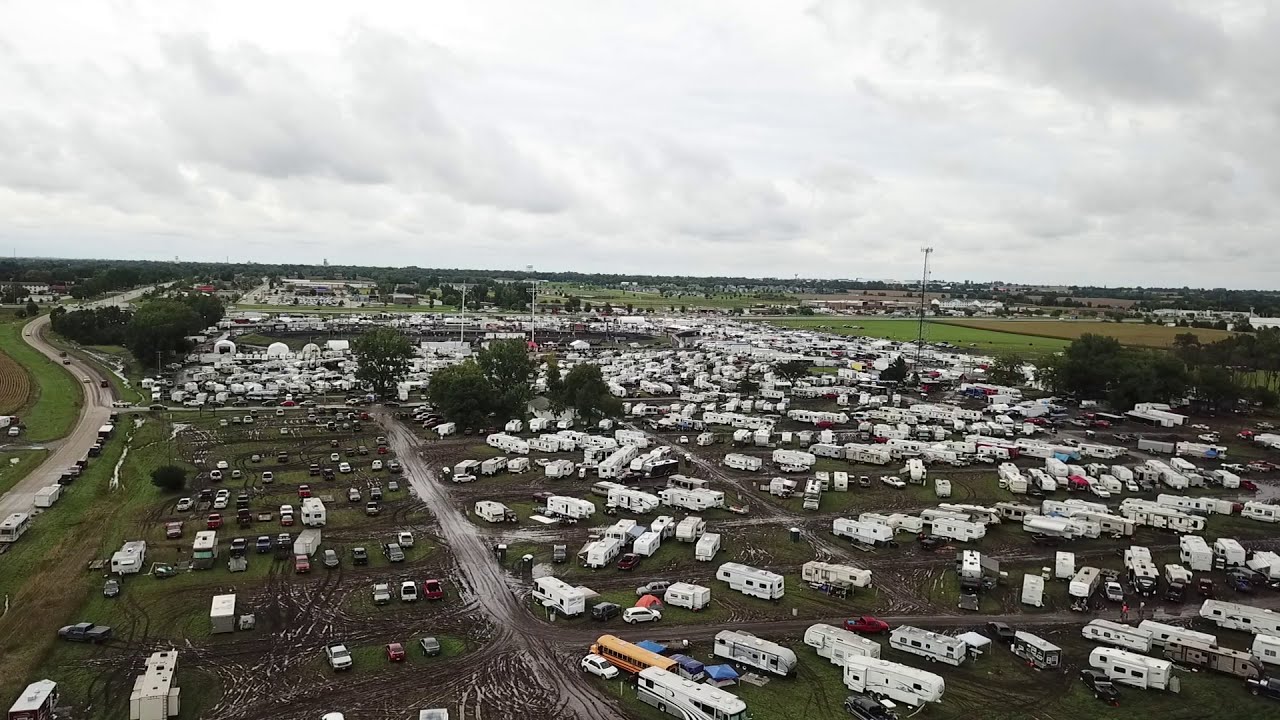This aerial color photograph captures a sprawling outdoor parking area or campsite, predominantly filled with hundreds of white RVs and campers dispersed throughout a vast, grassy expanse. The campers are arranged in rows primarily on the right side, with some vehicles scattered on the bottom left. Dirt paths crisscross the green grass, contributing to a muddy appearance where vehicles have traversed. To the left, a faintly visible road runs through the scene, while the background showcases distant buildings and fields bordering the edge of a green pasture. The landscape orientation emphasizes the overwhelming number of trailers hitched to cars, standing out starkly against the green grass and brown pathways. The overcast sky occupies the upper portion of the image, dominated by thick, fluffy clouds that cast a gray, almost wet, ambiance over the scene, underscoring the realistic, representational style of this drone photograph.